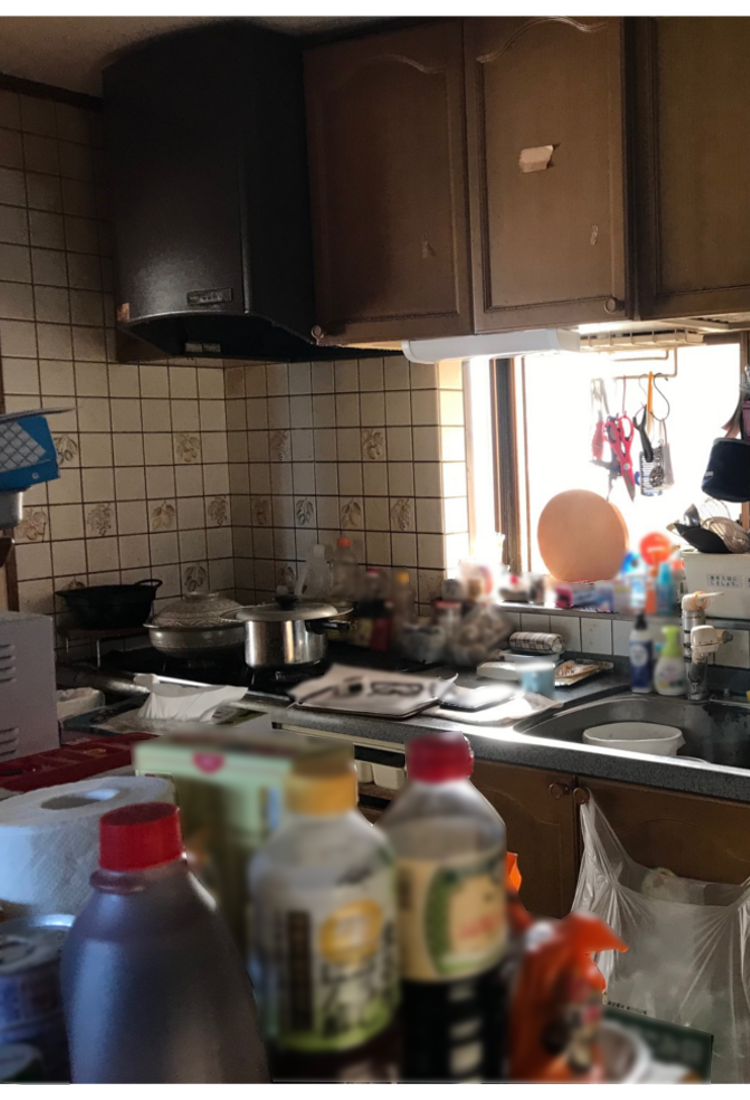This image depicts a cluttered kitchen with dark brown wooden cabinets overhead and walls entirely covered in white tiles. Dominating the center is a stovetop with a range hood positioned unusually high above it. The stovetop holds a wok and a pot, both covered, with paper towels and a spoon placed on top. Below the pots, there's an oven door. To the left, a sink houses a plastic bucket and a bottle of hand soap. Directly in front of the sink, wooden drawers have a plastic bag tied to one of their handles. A large window above the sink floods the space with sunlight, although it is cluttered with various decorative items. In the foreground, a surface is littered with several bottles, possibly ginger ale and drain cleaner. The entire kitchen appears overwhelmingly messy, with no available counter space, suggesting either disarray or a recent move into the home.